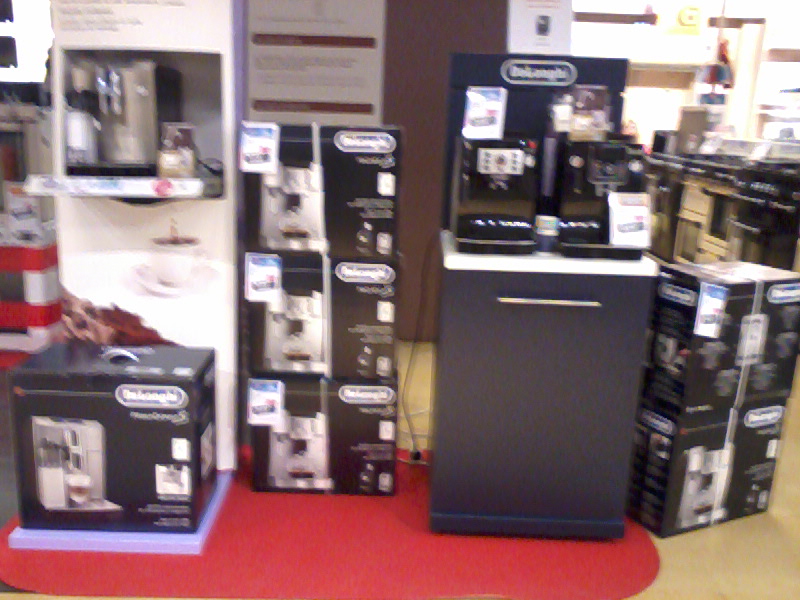The image depicts a blurry aisle within an electronics or home improvement store, possibly resembling a Home Depot. Central in the photograph, slightly to the right, is a black and gray piece of machinery with buttons that glow, likely a coffee maker based on the visible cup of coffee image on the display. Surrounding this machinery, there are stacks of black boxes, prominently featuring logos with elongated oval shapes containing the company’s name. Additional boxes are arranged on the left and right sides of the aisle. The setup rests on a round red carpet, contrasting with the stonish or polished yellow flooring. The walls and shelves in the background are white and brown, some shelves accented with red trim. Above the boxes, blurred poster boards with descriptions hint at the store's commercial setting, though no text is readable. Another aisle intersects perpendicularly, adding depth to the scene.